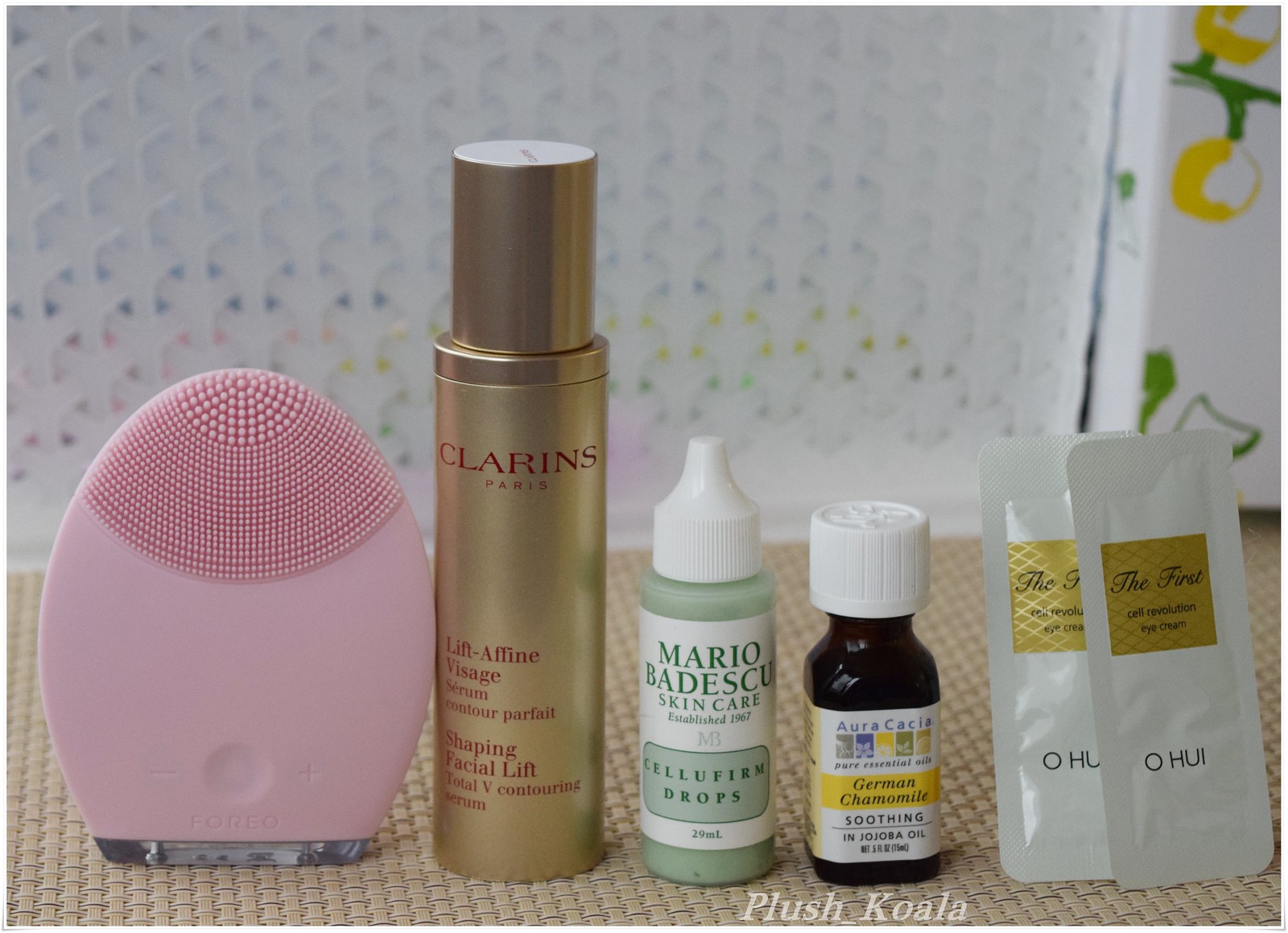In this vibrant photograph of skincare products, the backdrop features a colorful array of textiles or tiles with varying shades of yellow, green, blue, and pink, adding a lively aesthetic. Positioned to the side is a box top adorned with small, colorful shapes in yellow and green.

The foreground showcases an assortment of skincare items. First, a device resembling an Oreo with positive and negative symbols, possibly a face scrubber. Next is a pink, egg-shaped item with ruffled edges, likely another skincare tool.

A collection of bottles and serum drops include a gold bottle labeled "Clarins Paris - Shaping Visual Lift Total V Contouring Serum," and a green bottle called "Madera Serum Drops," which seems to be for topical application. Additionally, there’s a small bottle of “Soothing Java Oil” with German Chamomile.

Completing the ensemble are two packets of eye creams branded "O-HUI," packaged in distinctive gold and white. This photograph artfully combines a colorful background with an array of diverse and intriguing skincare products.